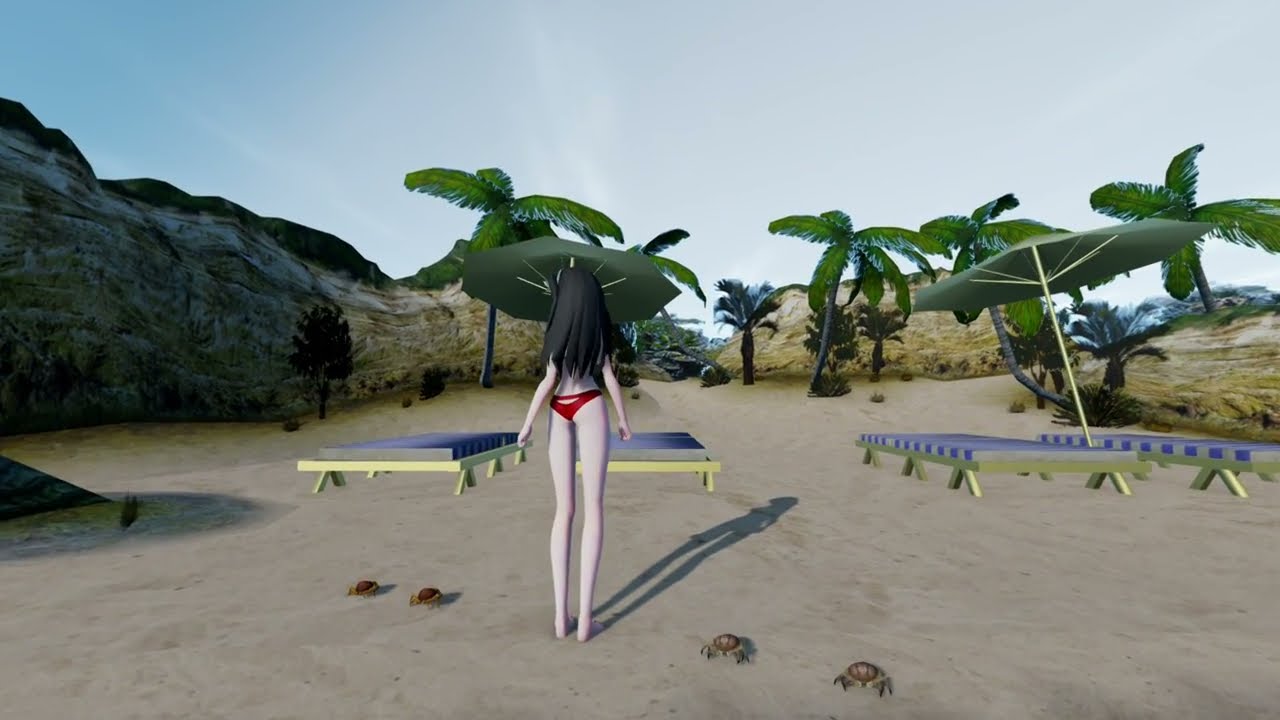In this AI-generated beach scene, a fair-skinned woman with long, dark hair stands at the center, her back to the viewer, wearing only red bikini bottoms as her hair cascades almost to her waist. Four crabs are scattered around her feet, two on either side. In front of her are four pixelated lounge chairs with purple wooden slats and brown bases, set up under two green umbrellas. The sandy beach is fringed with seven or eight palm trees scattered throughout the rocky valley. Rocky crags frame the scene on the left and right, leading to a distant view of the sea on the horizon. The sky above is a gradient of light blue, blending into misty white clouds, completing the serene yet distinctly computer-generated landscape.